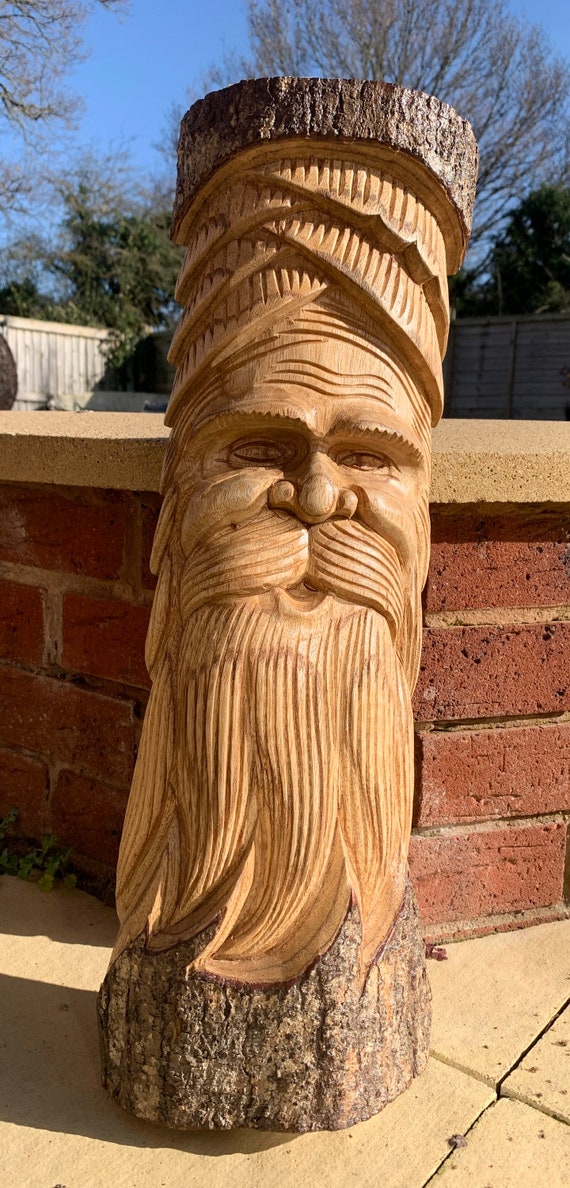This photo showcases a highly detailed wooden carving made from a large tree trunk, approximately four feet tall. The intricately carved face depicts an older man with a long, flowing mustache and beard, which splits into multiple points, suggesting a wave-like motion. His well-fed appearance is accentuated by the three pronounced creases on his forehead, detailed eyebrows, eyes, and a wide-set nose. The man's slightly agape mouth gives the impression that he is speaking, adding a sense of life to the carving. The sculpture is positioned at the corner of a short brick wall, which is topped with concrete and situated near a sidewalk. Some green vegetation peeks out next to the wall, and a white planter is visible on the far left of the image. Behind the carving, the background features a blue sky, a fence, and some trees, contributing to the serene outdoor setting.